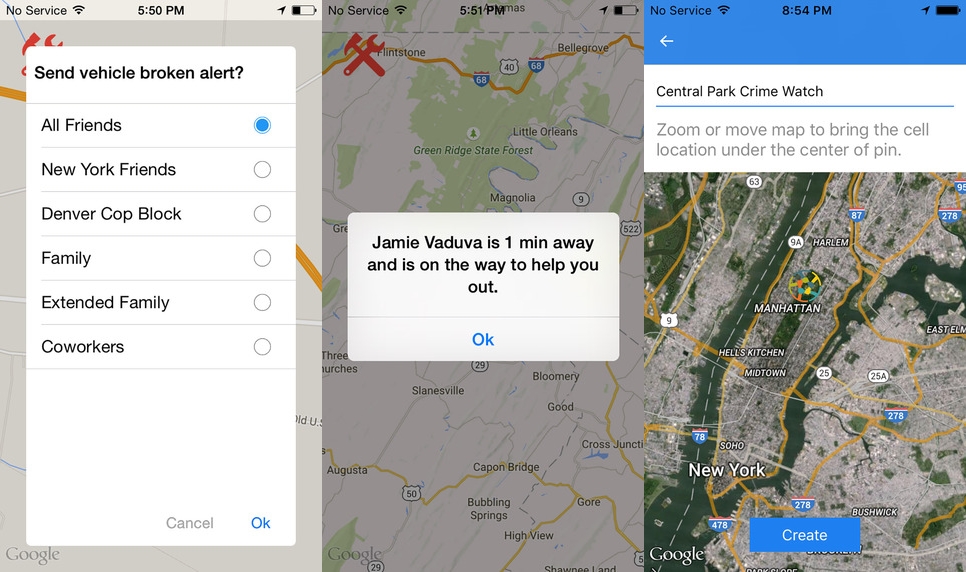Caption: 

The image comprises three overlapping screenshots taken from a mobile phone, each displaying a map interface. At the top of the screen, a notification banner reads "Send Vehicle Broken Alert," with options labeled "All Friends," "New York Friends," "Denver Cop Block," "Family," "Extended Family," and "Coworkers." The user has selected the "All Friends" option. Below this, a notification indicates that "Jamie Vagiba is one minute away and is on the way to help you."

The map in the background is detailed, featuring orange lines representing roadways, green areas signifying parks or open spaces, and various city names and regions, with a clear focus on Manhattan, New York. Central Park is prominently mentioned within the map interface.

At the top of one of the screenshots, a blue rectangle houses a white arrow pointing to the left, adjacent to a white rectangular banner stating "Central Park Crime Watch." Instructions below prompt the user to zoom or move the map to align the cell location with the center of a pin. The bottom portion of the screen displays a blue rectangular button labeled "Create," intended for creating new alerts or entries.